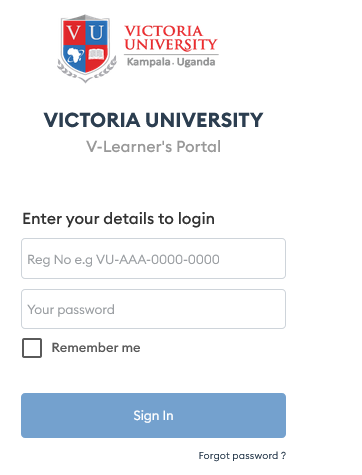The sign-in page is designed for the Victoria University V-Learners Portal, associated with Victoria University in Kampala, Uganda. Centered at the very top of the page is the title "Victoria University Kampala, Uganda," accompanied on its left by the university's logo. The logo resembles a coat of arms featuring red and blue squares. The top squares contain the letters "BU," while the bottom squares display an outline of the African continent and an open textbook.

Below the header, the text "Victoria University V-Learners Portal" is prominently displayed. Directly beneath this, the page instructs users to "Enter your details to log in." Two text fields are provided: the first one is labeled for "Registration number" with an example format "e.g., vu-aaa-0000-0000," indicating the required format for the school registration number. The second text field is designated for "Password."

There is a checkbox with the label "Remember me" next to it, allowing users to save their login details for future sessions. A large blue button labeled "Sign in" is prominently placed below the text fields. Additionally, in the lower right corner of the page, there is a link titled "Forgot password," providing users with an option to recover their login credentials if needed.